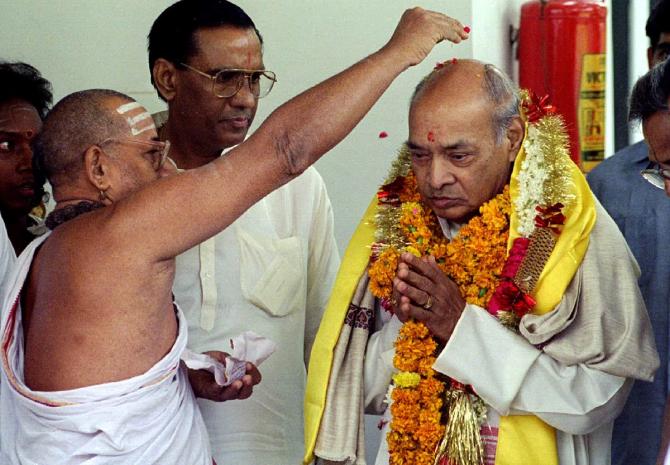The image depicts an older, likely 1970s or 1980s, Indian religious ceremony featuring an older man who appears to be a priest. He is distinguished by a red dot on his forehead and garlands of flowers, along with a yellow flower-filled scarf around his neck. This priest is wearing a white robe and is in a prayerful stance, possibly being blessed. To his right, another man in a button-up shirt and glasses participates in the ritual. A bald, glasses-wearing religious figure with white stripes on his forehead and clad in a robe, sprinkles red flower petals onto the priest's head. Other attendees can be seen in the background, standing near a white wall and a cylindrical fire extinguisher. The solemn ceremony is characterized by the ritual of flower pouring, with both the giver and receiver displaying reverence during the blessing.